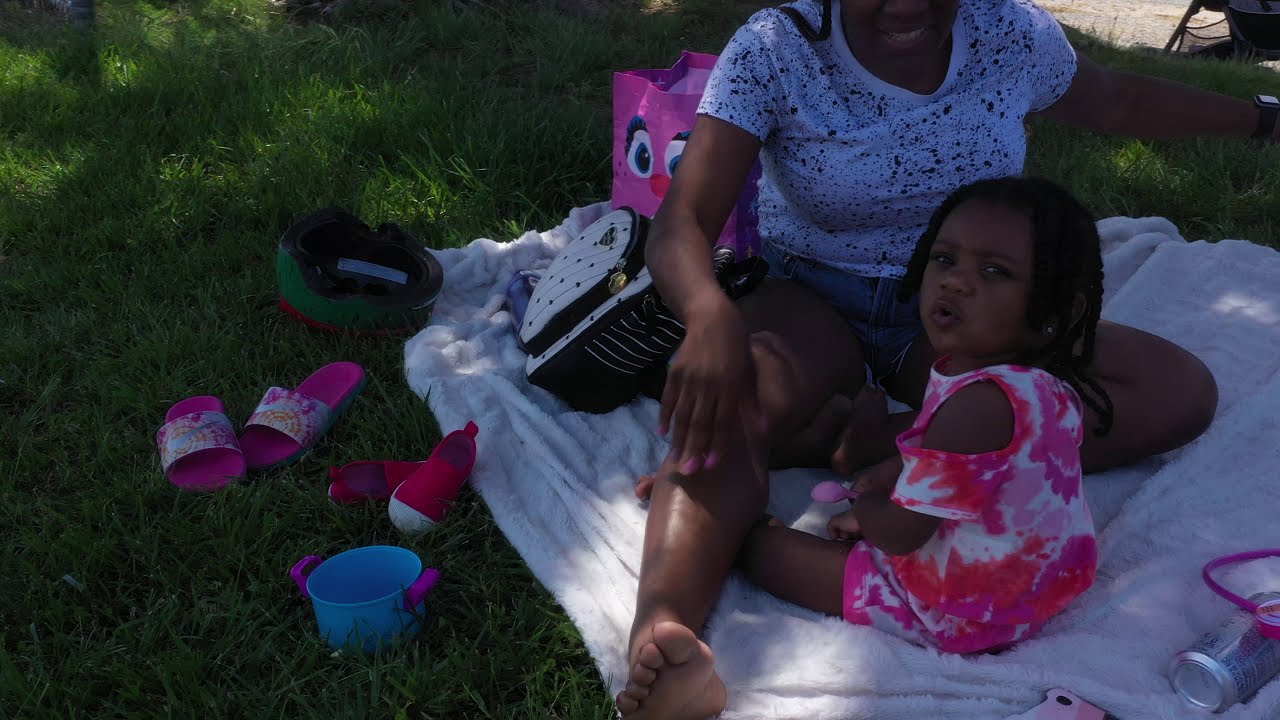In this detailed photograph, we see an adult woman and a little girl sitting on a white blanket spread over lush green grass. The area is mostly shaded, possibly by a tree, with some patches of sunlight filtering through. The woman, whose head is cropped out of the image, is wearing a white t-shirt splattered with black and blue shorts. She has her legs stretched out, revealing a light-skinned sole. In front of her sits a dark-skinned little girl in a cornrow hairstyle, wearing a pink dress with a tie-dye reddish-white and purple pattern, and short-sleeved pants. The girl is facing her mother but has turned her head to look directly at the camera. 

Around them, we can spot various items indicating a casual outdoor setting, perhaps a picnic. There's a small blue bucket with purple handles next to the blanket and a pair of purple sandals. To the left, an upside-down green helmet lies on the grass, hinting someone may have biked to the location. Behind the woman, a purple bag with eyes and a pink nose is visible, along with a black and white shoulder bag at her side. Additionally, a soda can rests in the lower right portion of the blanket. The scene is vibrant, featuring an array of colors: light blue, pink, orange, white, magenta, brown, red, black, gray, silver, dark green, and beige. The photograph captures a serene moment in a shady, outdoor picnic setting, emphasizing the relaxed and playful atmosphere.